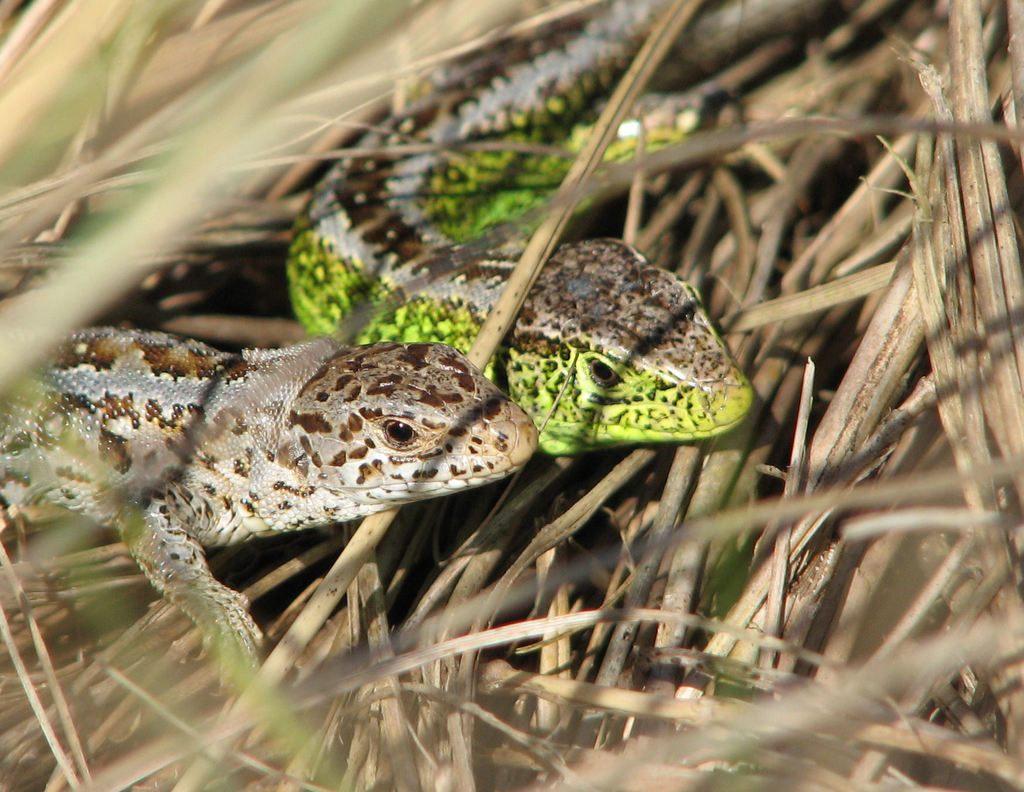The image captures a detailed close-up of an overgrown, dry grassy area illuminated with sharp, angular shadows cast by the straw-like blades. At the center of this scene, two reptiles are visible. One is a vibrant green and brown lizard, the green being particularly intense and eye-catching, while the other is silvery light brown and white, featuring brown spots and distinctly recognizable scales along its back. Both reptiles are facing towards the right with their closed mouths and dark eyes, their heads bowed close together, almost touching in what appears to be a wary interaction possibly reflecting a parent-offspring relationship given their different colors and sizes. The overall quality of the photograph is high, highlighting the texture of the dried grass and the intricate details of the lizards' scales and forms. The composition measures approximately 9 inches in width by 8 inches in height and contains just the natural elements without any additional text.